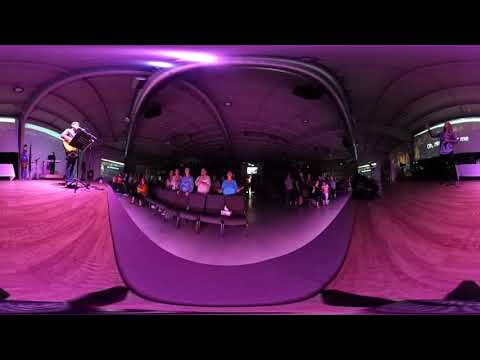This panoramic shot captures a dynamic scene with noticeable distortion, placing us in what seems like an indoor concert or church venue. The camera appears positioned high up on a stage, revealing a wide view of the event. On the left side of the image, a man stands next to a music stand, holding a guitar and seemingly singing into a microphone. The audience, occupying theater-style rows of chairs, are standing and clapping, perhaps giving a standing ovation. The central and right sections of the stage feature a woman gesturing or possibly using sign language, engaging with the crowd. The scene is bathed in a purplish-red hue, adding to the vibrant atmosphere. The ceiling curves above, framing the scene that blends musical performance with an active congregation, comprising mostly middle-aged individuals.